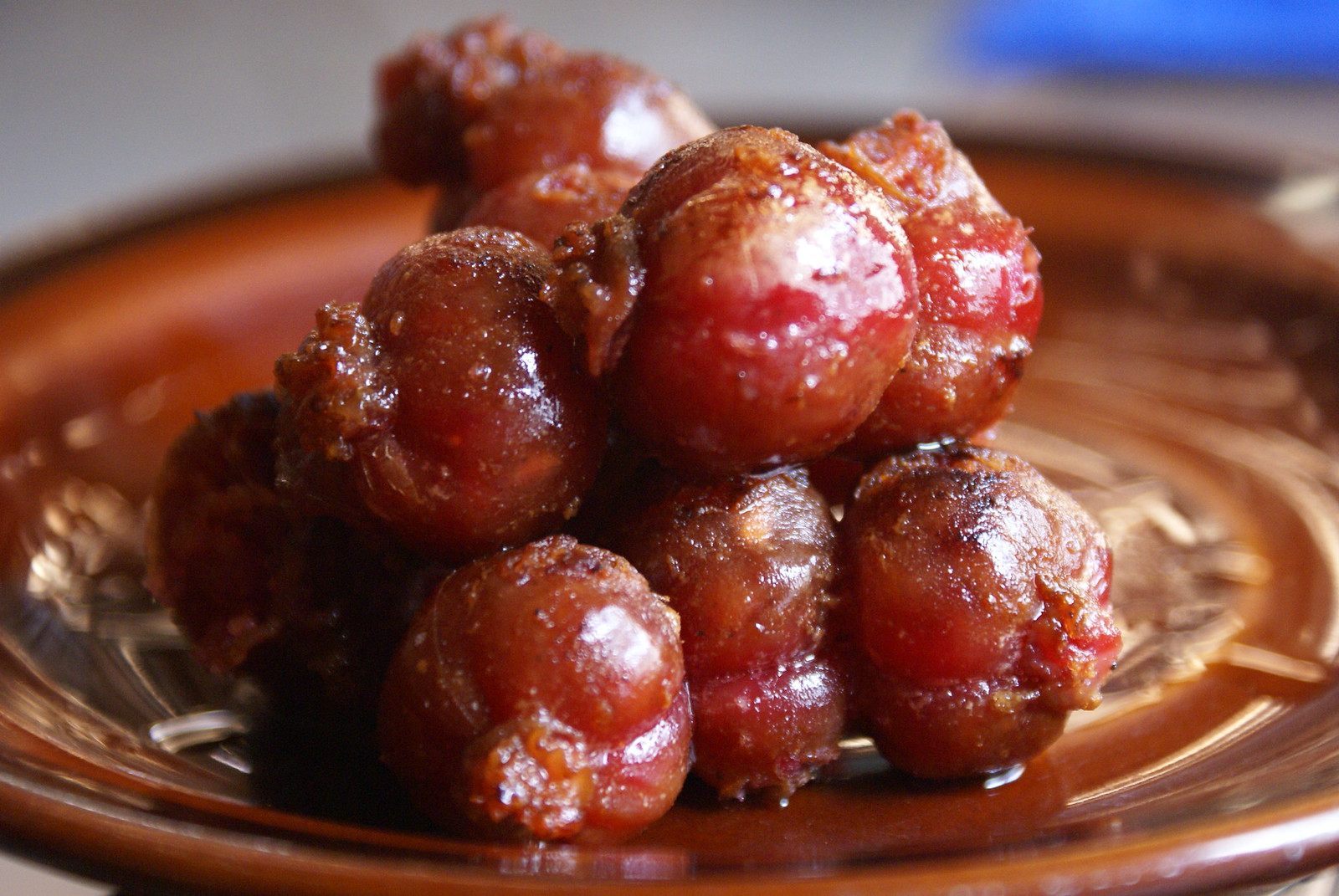In the image, a delectable serving of Chorizo de Cebu is showcased on a glossy, ceramic brown plate with a thick glaze. The chorizo pieces are small, sphere-like shapes resembling candied cherries, and are neatly stacked in the center, exhibiting a rich red-brown color with a glistening glaze. The entire arrangement is highlighted by soft yellow lighting, enhancing the appetizing allure of the chorizo. The background is a neutral gray, contrasting with the vibrant colors of the dish. Notably, a bright blue, unidentified object is partially visible in the top right corner, adding an intriguing element to the otherwise minimalistic setting.